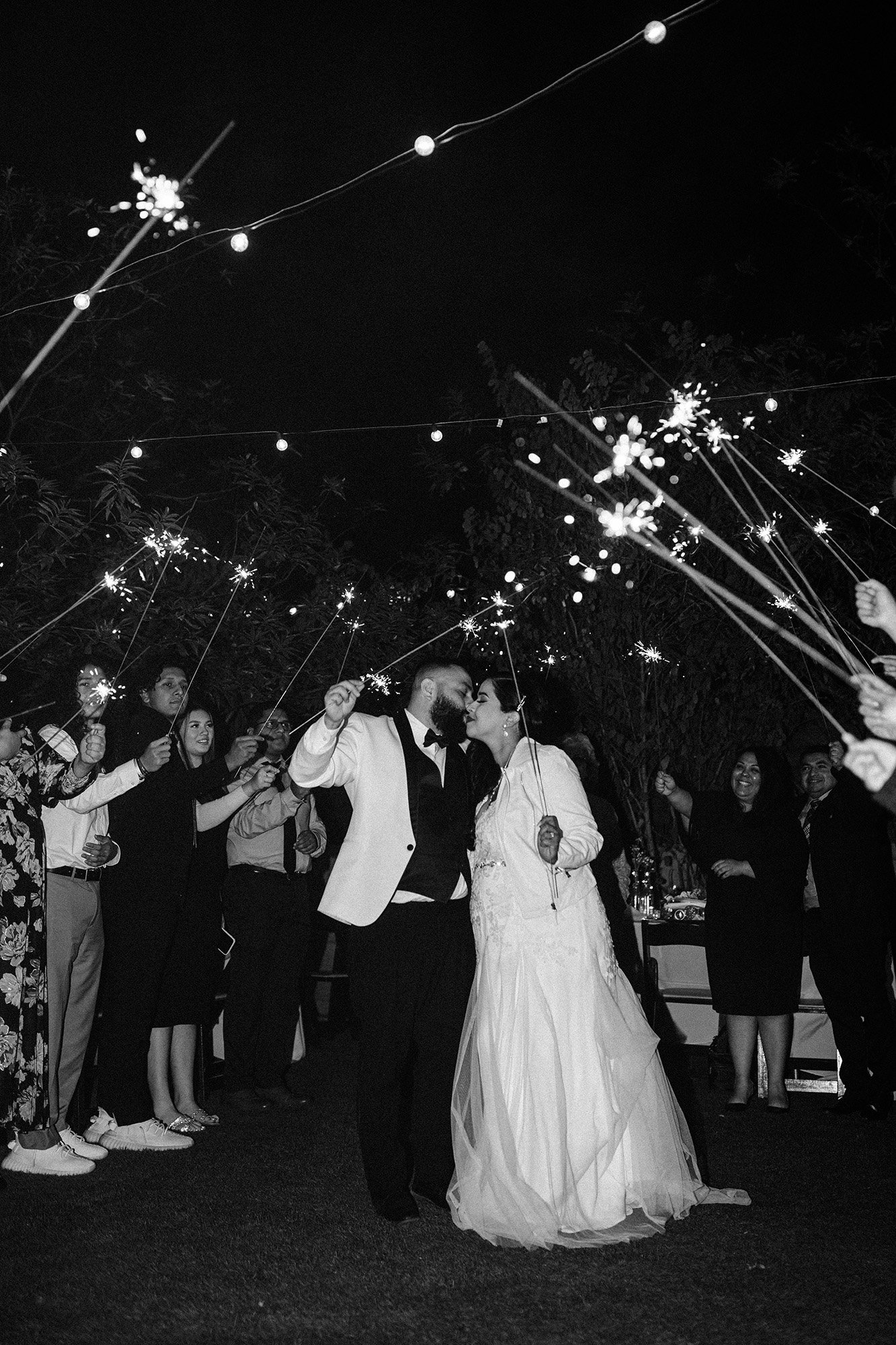In this black and white photograph, an intimate moment of a wedding celebration is captured beautifully. At the center, the bride and groom share a kiss under the night sky. The groom, bearded and donned in a white jacket, black vest and bow tie, black pants, embraces his bride. The bride, dressed in a long, lacy white dress with a voluminous, princess-like appearance, exudes grace and elegance. Her noticeable baby bump adds to the charm of the moment. The couple holds large sparklers that touch each other, illuminating their faces and the joy they share. Encircling them, their guests, all in formal yet casual attire, hold up sparklers triumphantly, creating a canopy of light. String light bulbs and tree leaves in the background hint at an outdoor setting, enhancing the romantic ambiance. The guests smile warmly, sharing the couple's happiness, but the bride and groom seem blissfully unaware of anyone else, lost in their own world.